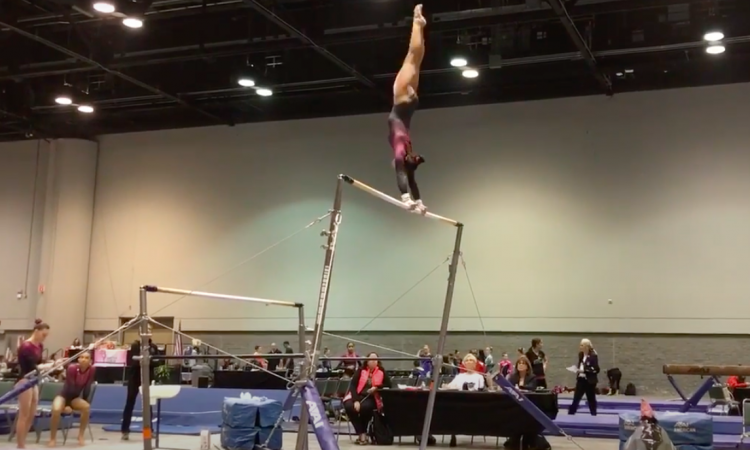In a towering gymnasium with high ceilings illuminated by fluorescent lights, a striking image captures a gymnast mid-routine on the uneven bars. She is perfectly vertical on the top bar, her body stretched into a flawless handstand with her arms gripping the bar and her legs pointing straight towards the ceiling. The gymnast, identifiable by her black long-sleeve leotard adorned with maroon detailing, appears to have brown hair. The gym's floor is lined with blue mats, and in the background, balance beams and additional gymnastic equipment can be seen. There are two judges' tables, one to the back left and one directly in front of the bars, both surrounded by people with papers and clipboards, indicating a competitive event. Teammates or fellow competitors in matching leotards stand just to the left of the lower bar, observing her performance. The gym's walls feature a stark contrast, with white upper sections and dark gray lower sections, further emphasizing the gymnast's poised and powerful presence against this dynamic backdrop.